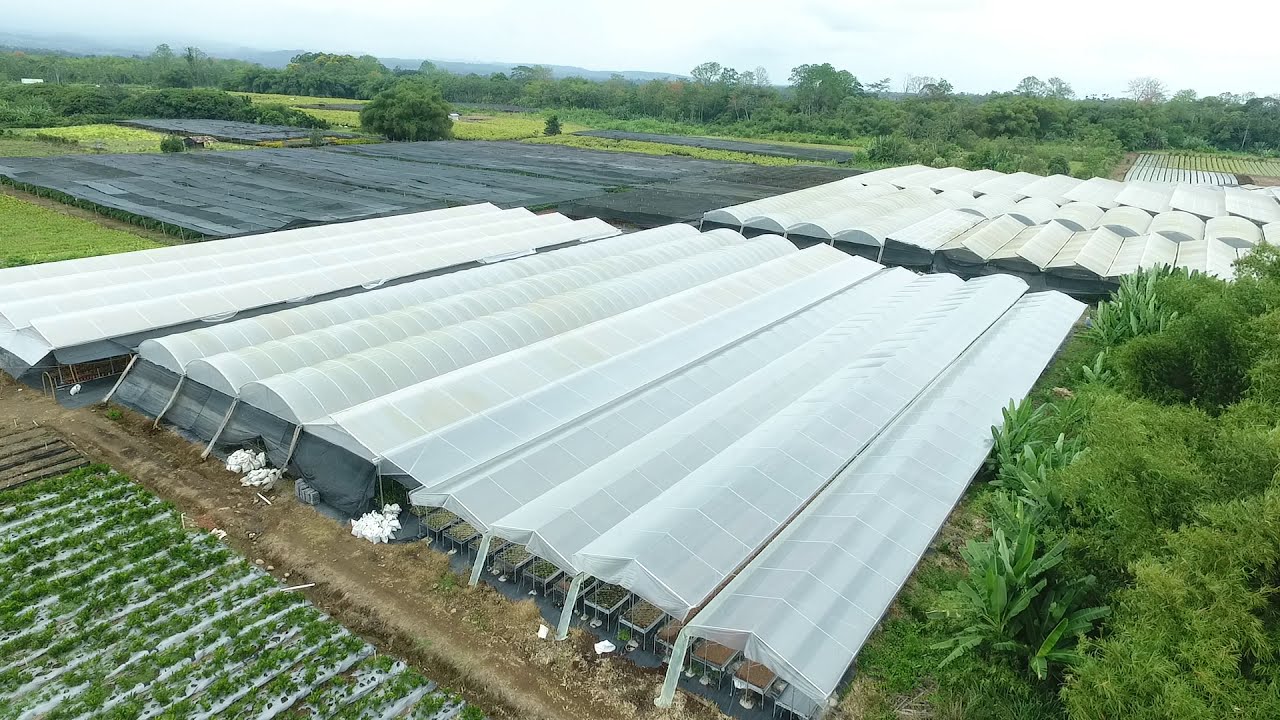This is a horizontally aligned, overhead photograph taken during a slightly overcast day. The image captures a large agricultural area with numerous long, rectangular greenhouses and fields. The greenhouses, with white or clear tops, run diagonally from the lower left to the upper right, totaling around 13 in the forefront, with additional rows visible in the background. Some of these structures have sides that are open, while others are covered with black tarps. In front of the greenhouses, a dirt path separates them from a field with rows covered in white material, likely for crop growth. Raised beds with various produce can be seen growing under the transparent tops of the greenhouses. The lower right-hand corner of the picture features a dense area of trees and natural foliage, while the upper part of the image is framed with more trees running from left to right. The sky and distant mountains are faintly visible, adding to the picturesque yet functional landscape. The surrounding area appears largely uninhabited, with no signs of homes, vehicles, or people, emphasizing the focus on agricultural production.